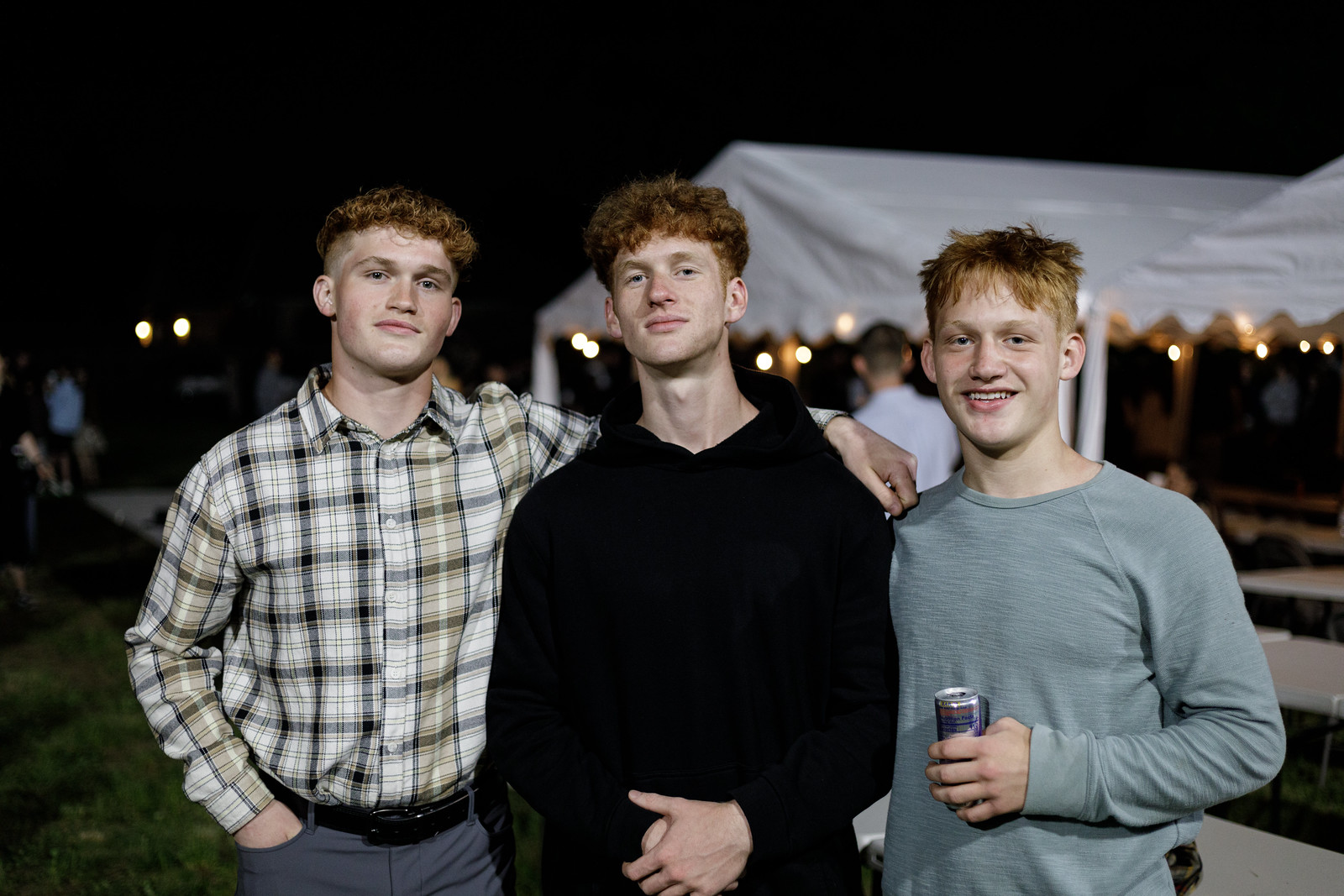In this nighttime outdoor photograph, three young men, possibly brothers due to their shared reddish-auburn hair, stand together in front of a white tent supported by a white awning and poles. At the far left, the first man sports a black and gold plaid shirt paired with blue pants and a black belt. His hair is curly with shaved sides, styled into a voluminous top. The man in the middle, dressed in a black hoodie, has short hair on the sides with curly locks at the top, and he stands with a confident expression. The third man on the right, the shortest and seemingly the youngest, wears a blue-gray long-sleeve shirt and holds a Red Bull can. His straight red hair is spiked out and slightly messy. The dimly lit background features scattered people, white tables, and patches of grass, all enveloped in the darkness of night.